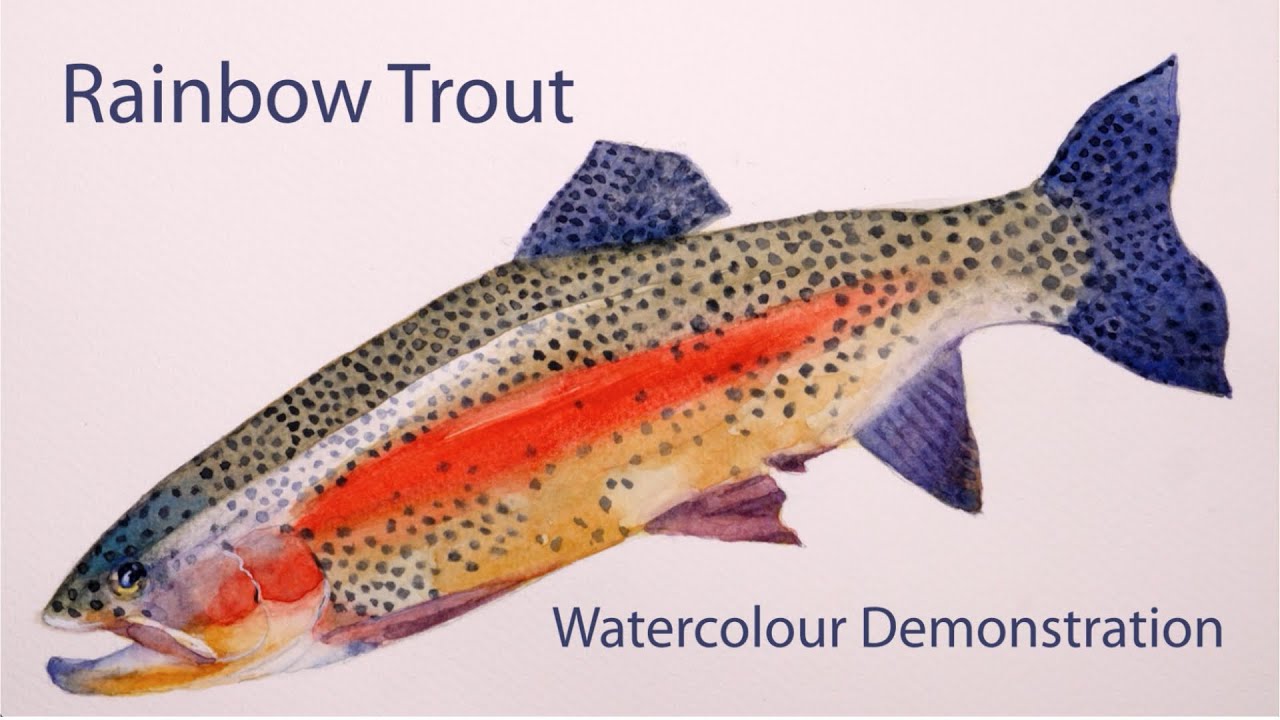The image showcases an exquisite watercolor painting of a rainbow trout set against a cream-colored background. This realistic and crisply detailed artwork captures the vibrant coloration of the trout, which features a prominent red stripe running horizontally along its tan body. The fish is peppered with numerous black dots and accents of blue, purple, yellow, and teal. Notably, the dorsal and tail fins display an indigo hue, while the side fins are a dark purplish color. Additional splashes of light and yellow are visible on the trout's jaw and side. The fish appears to be depicted with a slightly upward-curving mouth, giving it a subtly expressive look. In blue text, "Rainbow Trout" is labeled in the top left, and "Watercolor Demonstration" is written in the bottom right, suggesting that this image might be part of a tutorial or simply showcasing the final result of a detailed watercolor project. The fish is oriented with its mouth pointing to the bottom left corner and its tail to the top right. Overall, the artist has successfully rendered a lifelike and colorful depiction of the rainbow trout.